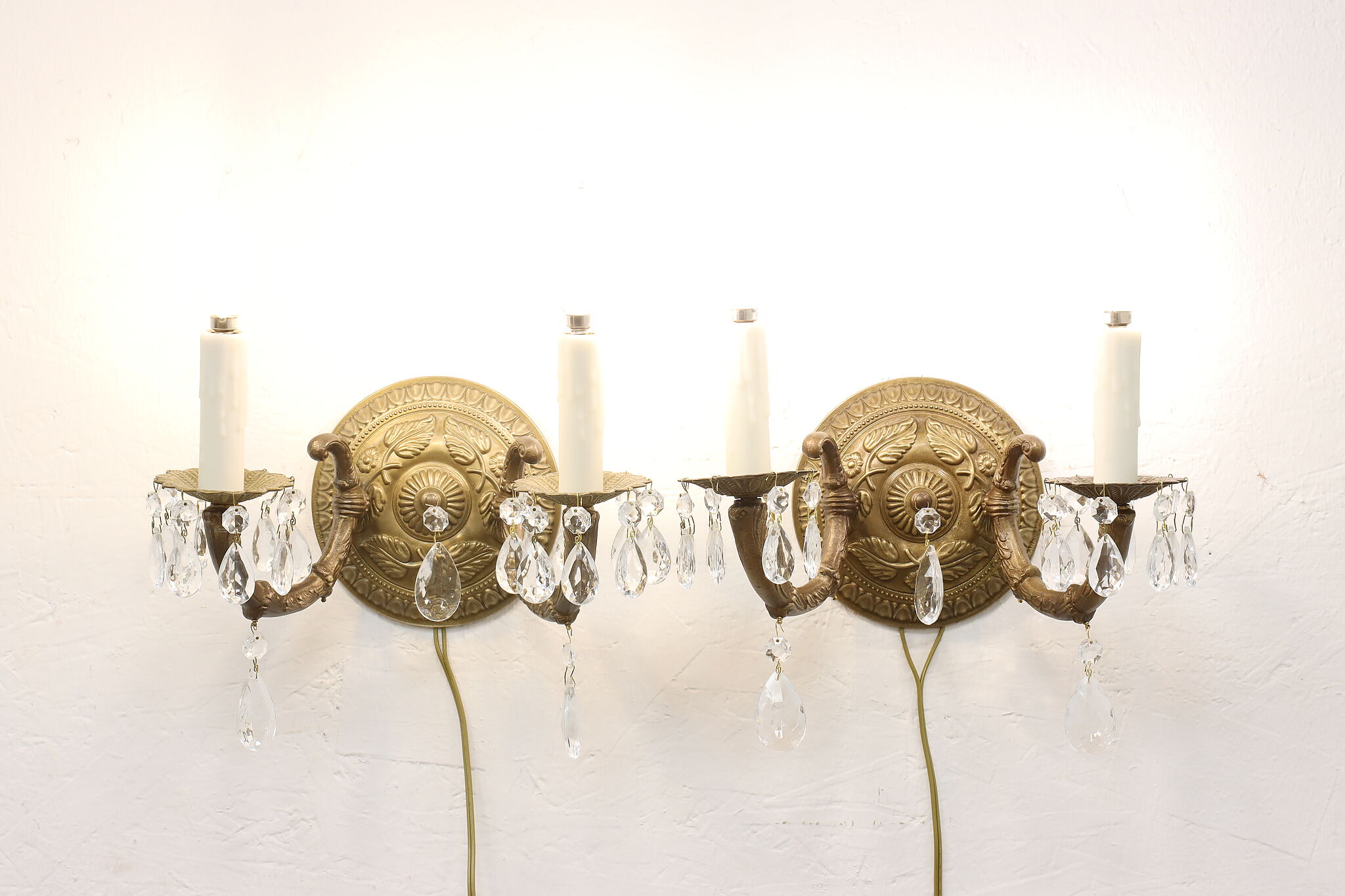The photograph, taken indoors, captures two identical, intricately designed candle sconces mounted side by side on a wall. The wall appears almost white with a subtle pink or purple cast near the edges. Each sconce features a central circular frame, about eight inches in diameter, made of light brownish metal, adorned with elaborate designs of leaves and flowers. Extending from the central circle are two gracefully arched arms ending in small trays that hold what look like white plastic candles, which emit a bright white light, creating an illuminated backdrop. Both sconces showcase beadwork, including a small hanging glass bead at the center, leading to a teardrop-shaped bead below. From the bottom of each sconce, wires emerge and converge, trailing down to the bottom of the photograph, hinting at an electrical connection powering the light source.